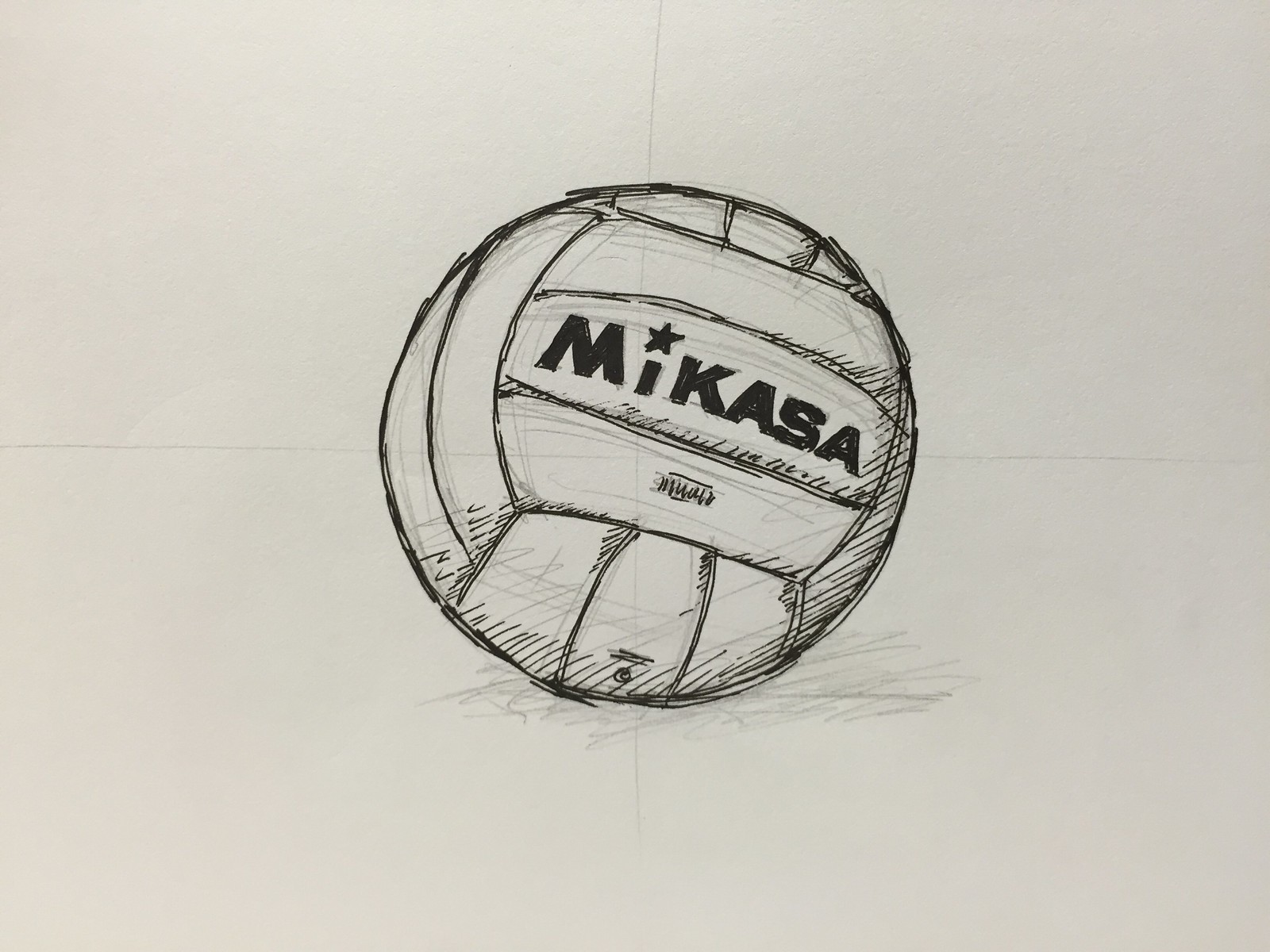The image showcases a detailed pencil drawing on a white, slightly grayish paper background. At the center of the image is a realistic depiction of a volleyball. The ball prominently features darkened, bold letters spelling "MIKASA," with a star replacing the dot above the letter "I". The volleyball is divided into distinct rectangular sections by both horizontal and vertical lines. Additional shading, composed of fine lines, adds depth and dimension primarily to the bottom and right portions of the ball. There is also a small square of shading directly beneath the "MIKASA" text. The entire composition is intersected by faint grayish lines that form a plus shape across the center of the paper. The attention to detail in the shading and line work lends a very realistic quality to the drawing.